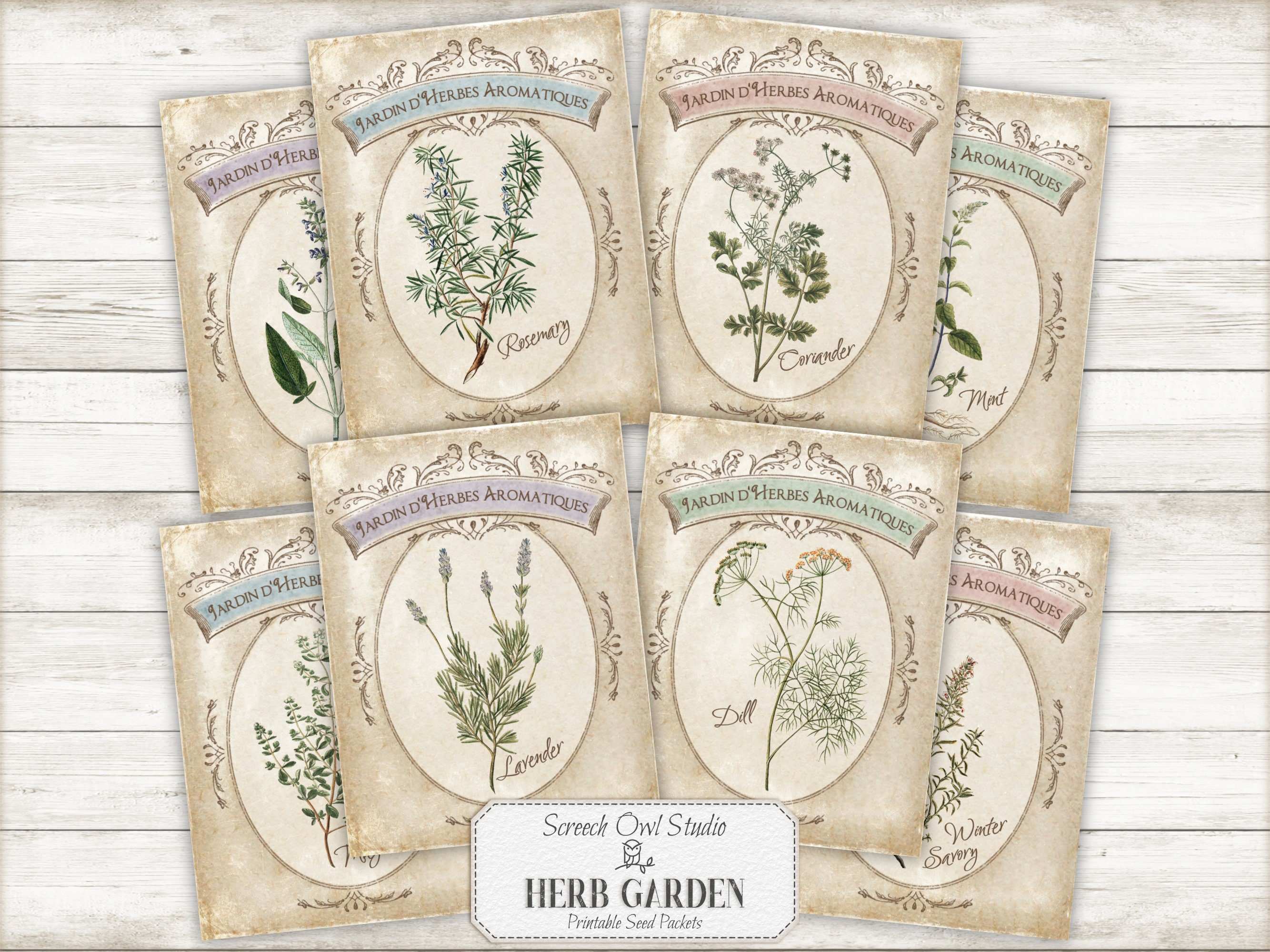This image features a well-arranged illustrative set of eight herb seed packets, portrayed in a light watercolor style with a tannish background. Each packet is adorned with a white oval center, showcasing a detailed, green watercolor depiction of the corresponding herb. The top and bottom rows both consist of four packets, with the second and third packets in each row slightly overlapping the first and fourth, creating a cohesive semi-circular fan layout.

The top row includes the following:

1. A partially cut-off packet labeled “Jardin d'herbe,” displaying a leafy green plant.
2. A packet labeled “Jardin d’herbe aromatique,” featuring an image of rosemary with the label inside an oval.
3. Another “Jardin d’herbe aromatique” packet displaying coriander in an oval.
4. The final packet in the top row shows mint within an oval.

The bottom row mirrors the top's organizational style:

1. A partially cut-off packet also labeled “Jardin d'herbe,” featuring a green plant.
2. A packet labeled “lavender,” showcasing purple lavender flowers or plants.
3. A packet for dill, with thin green leaves and possibly some flowers illustrated.
4. The last packet displays winter savory, depicted with spiky green plants or flowers.

At the bottom of the image, the label "Screech Owl Studio" accompanies a graphic of an owl along with the text "Herb Garden Printable Seed Packets," suggesting the source of the artwork. The earthy visual elements and precise arrangement of the seed packets evoke an organized and aesthetically pleasing image, perfect for gardening enthusiasts.